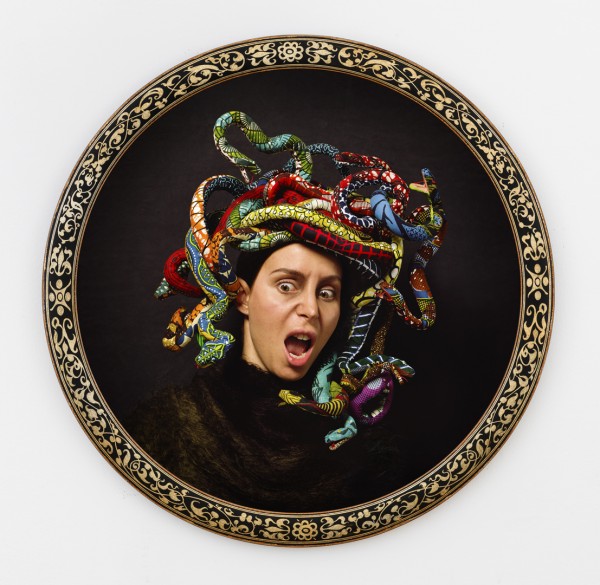This detailed and expressive artwork depicts a person in a round picture frame with an intricate gold-on-black design. The background of the picture is black, enhancing the dramatic focus on the central figure, who appears to be a woman. She is draped in a brown fur shawl around her neck, although another description suggests a dark green shirt covering her neck up to the chin. Her face is highly expressive, with her mouth open in a gasp of fright, and her eyes wide in alarm, conveying a mixture of surprise and horror.

Crowning her head, in place of hair, is a mass of multicolored snakes crafted from an array of materials and stuffing. These artificial snakes are adorned with wild, unrealistic patterns - paisleys, circles, and dots in vivid colors like greens, purples, reds, blues, yellows, oranges, and even pinks with whites. Each snake's mouth is ajar, revealing little tongues, reminiscent of the mythical character Medusa. This creative liberty with the snakes adds a fantastical element to the piece, capturing the viewer’s attention with its bold and surreal design. The entire artwork, currently set against a gray wall background, gives the impression of being an unusual and captivating piece of art, somewhere between a frightening vision and a fascinating spectacle.